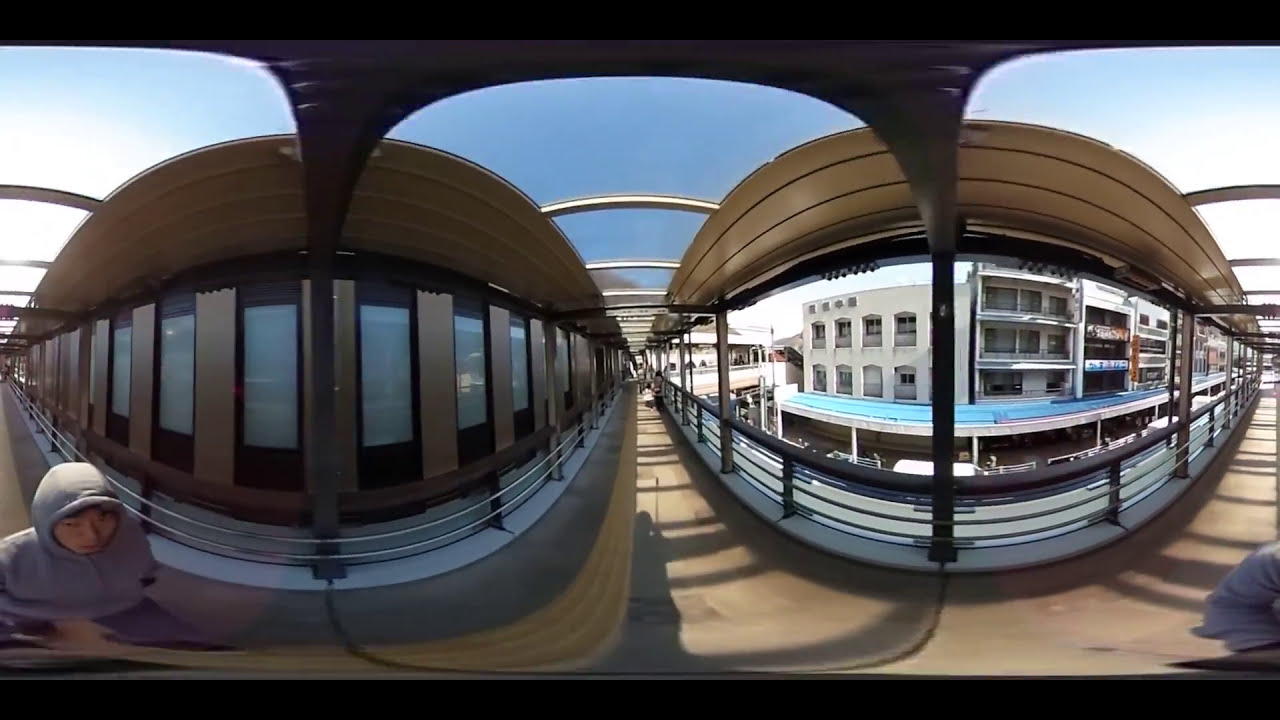The image captures an outdoor setting with a distinct curved perspective, making it appear as though the straight lines are bent into a circular pattern, akin to two large oval circles resembling eyes. The scene prominently features two buildings that create this eye-like illusion. The building on the right is off-white, approximately two stories high with a fence or gate around it, and has a parking structure beneath. The building on the left seems zoomed in, highlighting rectangular, blue-tinted windows. Three walkways are visible: one in the center, one to the right, and another to the left, contributing to the circular aesthetic. The sky is a clear daytime blue with some white clouds above the buildings. In the far left corner, a person wearing a gray hoodie, possibly with dark hair, is walking near the structures, appearing slightly distorted. The entire composition has a brown tint towards the top, enhancing the surreal, eye-like appearance of the buildings.